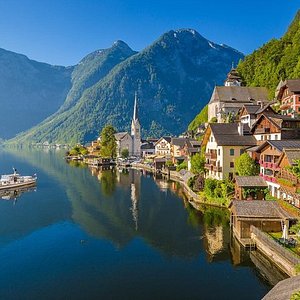The image captures an idyllic scene of the alpine village of Hallstatt, Austria, nestling against a mountainside by a tranquil lake. The village, situated on the right-hand side of the frame, features charming houses with dark red wood and white stone or stucco facades, topped with shingled roofs. Among these structures, a notable landmark is a small white church with a prominent steeple, standing near the shore. The lake, on the left side, mirrors the surrounding mountains, which range from lush light green to darker green hues in the distance, adding to the picturesque scenery. A white boat with a light brown underside floats on the clear, blue waters of the lake. The vibrant blue sky above completes the serene and breathtaking alpine landscape, underscored by green foliage and the stunning natural beauty of the mountains that envelop the village.